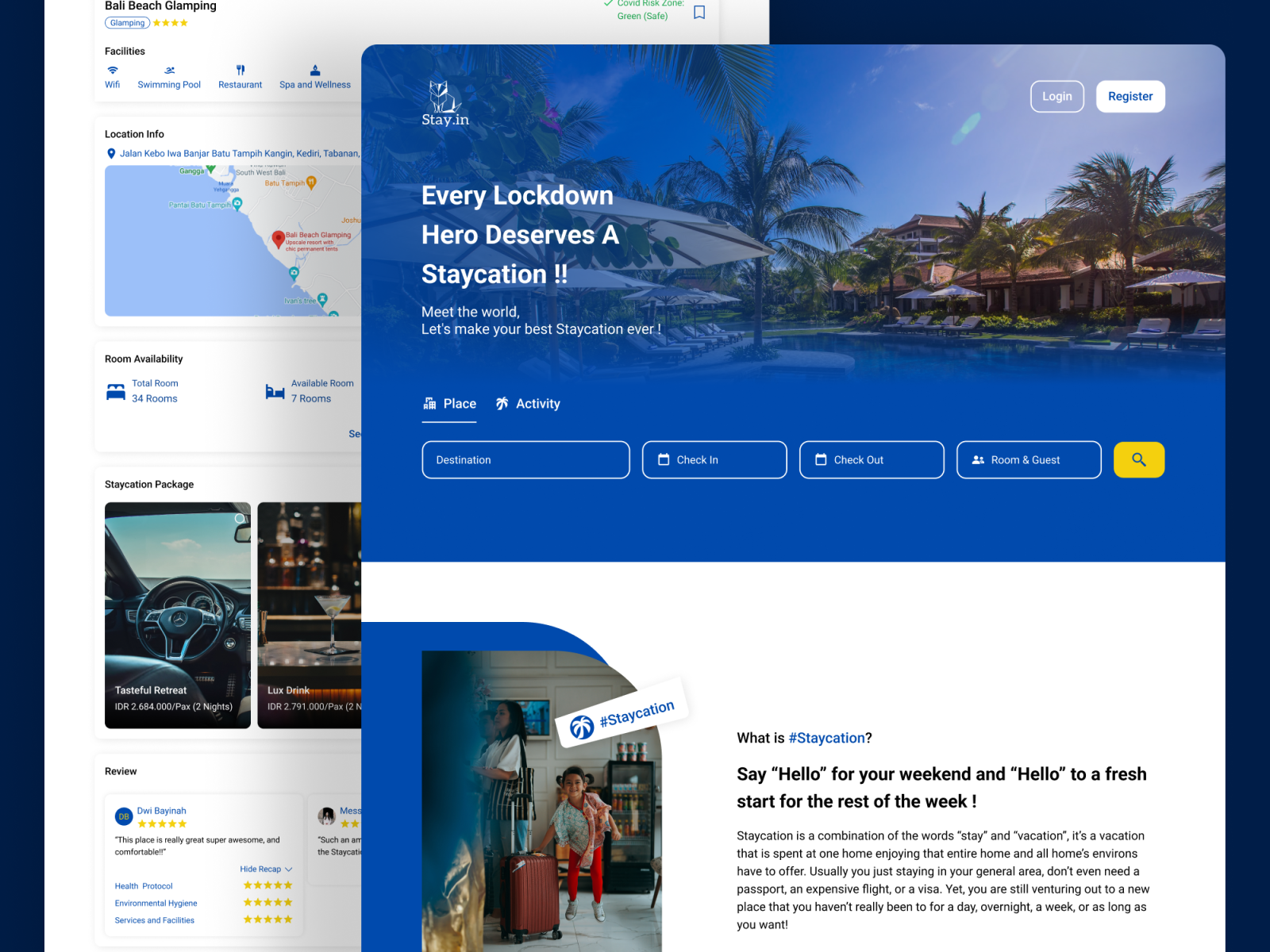### Detailed Caption for the Image:

In this image, prominently located in the top left corner, there is a text overlay that reads "Bali Beach Climbing." The visuals are split into two distinct sections, mimicking the appearance of two pages laid side by side. 

The left page serves as the background and features details about a Bali beach camping experience. Its topmost text indicates "Bali Beach Camping," rated with four stars. Beneath this, the amenities are listed: Wi-Fi, Swimming Pool, Restaurant, Spa, and Wellness. Further down, location details specify Tabanan, with information about room availability—34 total rooms, and 7 currently available. The section concludes with various staycation packages titled "Successful Retreat" and "Luxe Drink" along with a review by Duy Baena stating, "This place is really great, super awesome, and comfortable."

The right page, placed in the foreground, has a blue and white color scheme, forming the background for its content. The upper left corner displays "Stay In," while the upper right corner contains two interactive buttons labeled "Lock In" and "Register." The primary text below "Stay In" reads: "Every Lockdown Hero Deserves a Staycation. Meet the world, let's make your best staycation ever." Following this, there is a structured layout for input fields including "Place Activity," "Category," "Search by Destination," "Check-In," "Check-Out," and "Room and Guest," capped off with a bright yellow search bar.

At the bottom of the right page, explanatory text elaborates on the concept of a staycation: "What is Staycation? Say hello for your weekend and hello to a fresh start for the rest of the week. Staycation is a combination of the words 'Stay' and 'Vacation.' It's a vacation spent at one's home, enjoying the entire home or nearby homes and villas, negating the need for passports, expensive flights, or visas. It allows venturing out to new places in your local area for a day, overnight, a week, or as long as you desire." 

This comprehensive image offers a blend of information and functionality for those interested in a staycation, particularly highlighting the offerings of Bali Beach.